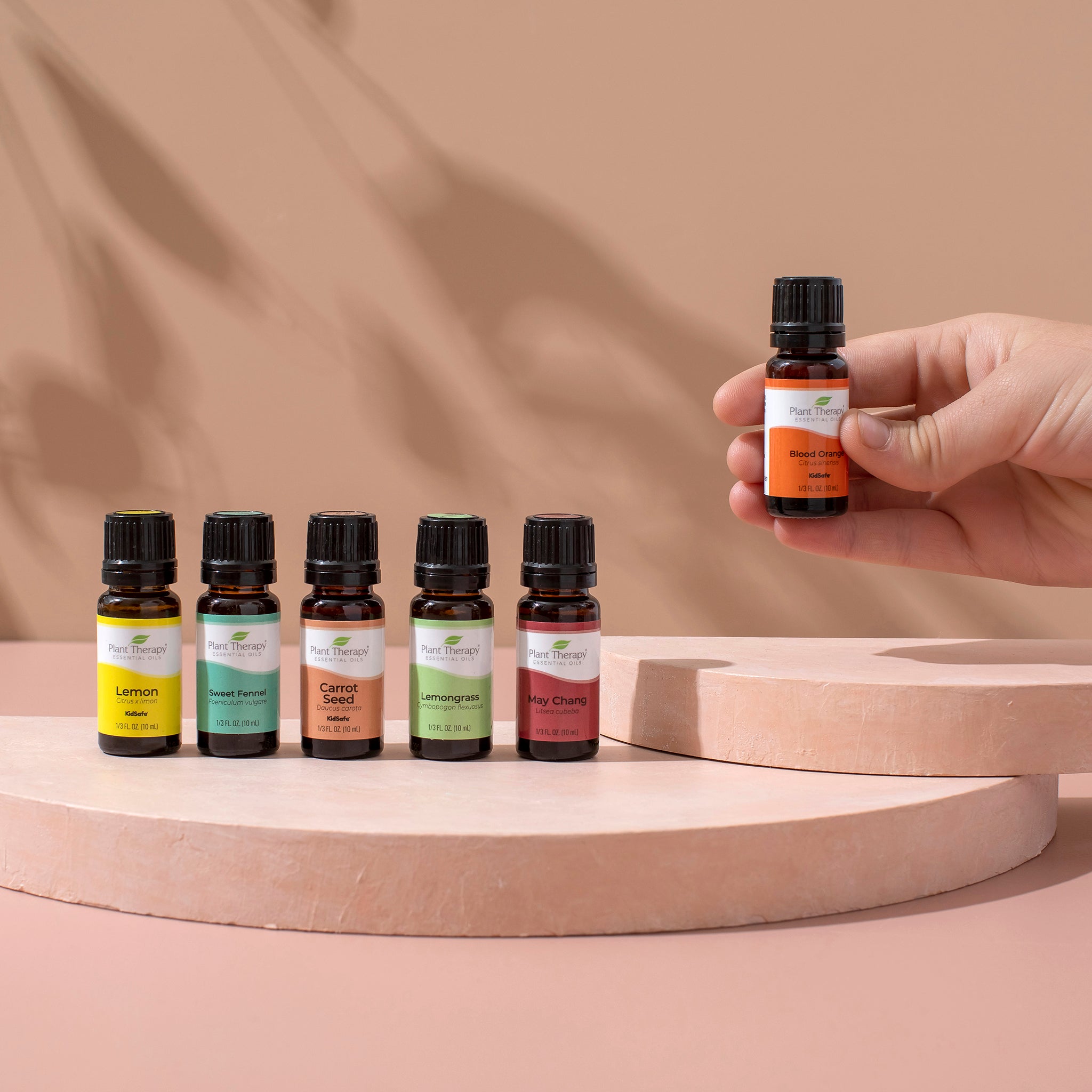The square photograph showcases an organized display of several small, round, dark amber glass vials with black, vertically grooved, twist-top caps, identified as essential oil bottles. A white hand emerges from the right middle side, holding one such vial, which has a distinctive orange and white label reading "Blood Orange." The labels on these bottles are color-coded and each bears the "Plant Therapy" logo, featuring a green leaf on a wavy white background. Arranged neatly on a small, circular, textured platform that is very light pink in color, the vials are lined up as follows: "Lemon" with a yellow and white label, "Sweet Fennel" with a green and white label, "Carrot Seed" with an orange and white label, "Lemongrass" with a green and white label, and "Mei Chang" with a red and white label. This platform is placed on a larger light pink counter or table. The background is a slightly blurry wall with streaks of light to medium brown hues, enhancing the focus on the bottles.